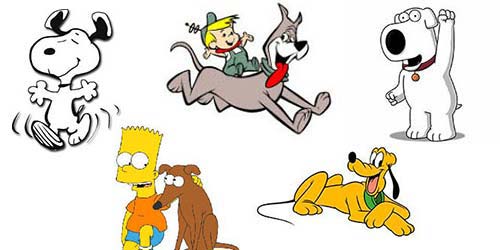This image showcases various beloved cartoon dogs on a white background, featuring five different characters. In the top left corner, Snoopy from "Charlie Brown" is joyously dancing with a smile; he's a white dog with black ears, a black collar, and a black nose. At the top center, there's a retro cartoon scene depicting a large gray dog with a red tongue hanging out, running while a small blonde child in a green hat and overalls rides on his back. The child is also accessorized with a red handkerchief. On the top right, Brian from "Family Guy" stands confidently with his left paw raised; he is an all-white dog with a big black nose, expressive white eyes, and a red collar adorned with a small tag. In the bottom left, Bart Simpson is shown kneeling and petting his sad-looking brown dog, who has a pointy nose and short ears. Bart, characterized by his spiky hair, red shirt, and blue shorts, appears concerned for his furry friend. Finally, in the bottom right, Goofy is lounging on his belly with his back legs slightly raised and his front legs crossed. He has black ears, a green collar, and his mouth is open, giving him a happy expression.